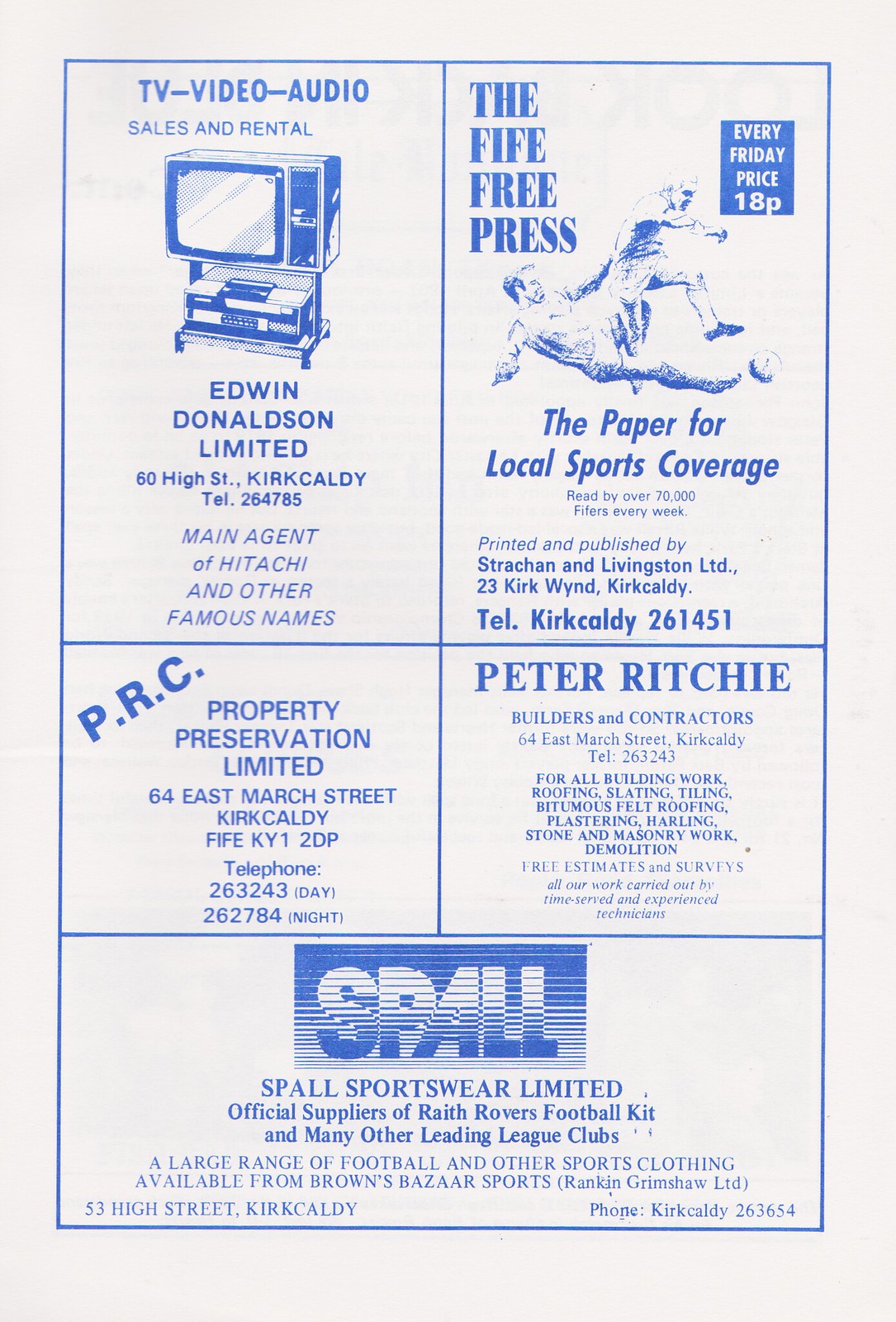This is a retro-style newspaper page featuring five distinct advertisements, all in shades of dark blue on off-white paper. In the upper left corner, an ad depicts a classic CRT TV on a stand, promoting "Edwin Donaldson Limited," a store located at 60 High Street, Kirkcaldy, specializing in TV, video, and audio sales and rentals. They are a main agent for Hitachi and other renowned brands. The upper right corner highlights "The Fife Free Press," a local newspaper celebrated for its comprehensive sports coverage, boasting a readership of over 70,000 Fifers weekly. It features an image of two soccer players mid-action, with one sliding for the ball and the other leaping. The bottom half of the page includes three additional ads: "PRC Property Preservation Limited," "Peter Ritchie Builders and Contractors," and "Spall Sportswear Limited," which is noted as the official supplier of the Wraith Rovers football kit and numerous other leading league clubs. The vintage aesthetic is accentuated by the detailed illustrations and classic typography.